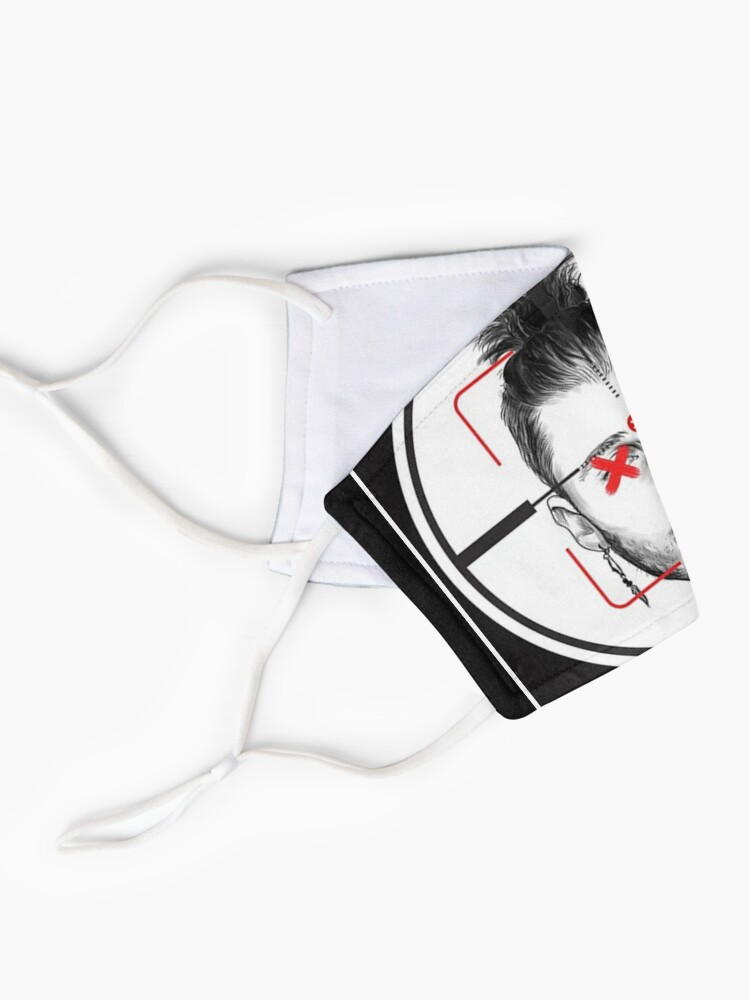The image depicts a fabric face mask commonly worn during the COVID-19 pandemic, prominently set against a stark white background. The mask is folded in half, revealing only one side. It features standard, knotted white elastic ear loops. The design on the mask is monochrome with dramatic red accents. Dominating the visible portion is a black-and-white illustration of a man's face, possibly resembling Machine Gun Kelly, centered within a series of concentric circles reminiscent of a gun's crosshairs or a bullseye. A distinctive red X slashes across one of his eyes, further emphasizing the target motif. Notably, the man's eye-catching features include a man bun and a long, dangling earring, adding a contemporary touch to the stark design. This may be a product photo or a design template showcasing the mask's graphic elements and aesthetic appeal.